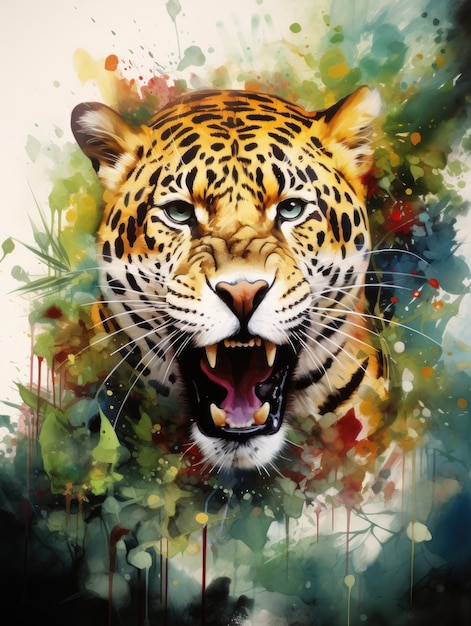The image features an intricate and skillfully rendered tiger's head, seemingly popping out at the viewer due to its dynamic details. The tiger, depicted from the neck up, is roaring fiercely with its mouth wide open, showcasing sharp fangs both on the upper and lower jaw. Its pointed ears, rounded at the tips, contribute to its lifelike appearance. The tiger's fur is adorned with black spots that transition into distinct stripes as they extend towards and down the neck. Its penetrating green eyes and orange nose enhance its intense expression. The background of the image complements the tiger’s ferocity with a splotchy graffiti-style array of colors, predominantly white with splashes of green and blue. This creates a vibrant and somewhat chaotic environment that frames the tiger perfectly, adding to the overall edgy and energetic vibe of the artwork.